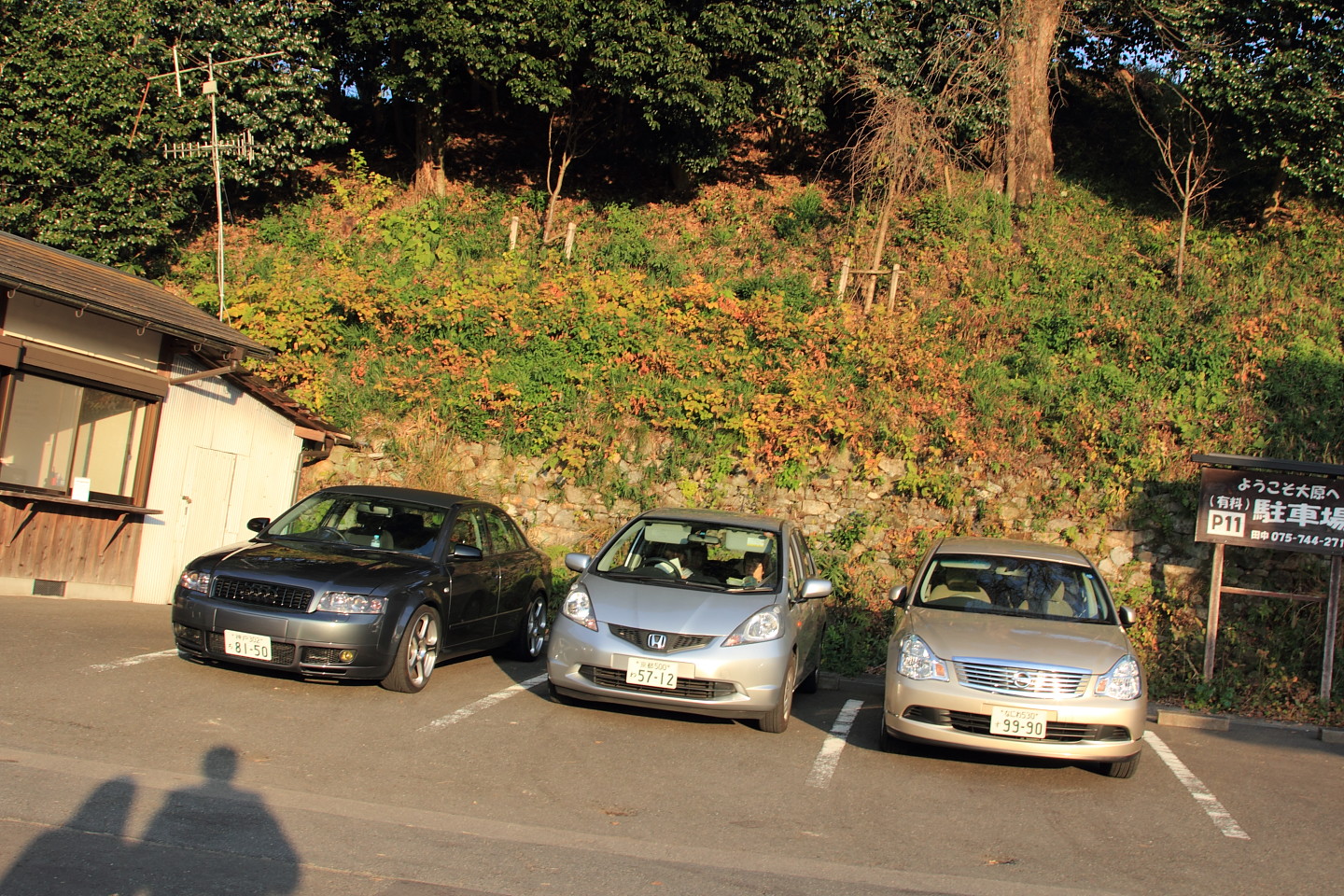This outdoor photograph captures a vividly detailed parking lot scene set against a green and brown hillside with a tree line and an array of bushes displaying varying shades of leaves. In the background, to the left, there is a small brown and white building featuring two windows on its brown side. Prominently, the parking lot in the foreground shows three sedans backed into parking spaces. On the left is a black car, followed by a silver Honda Accord in the center, occupied by two individuals reading books, and a light tan car on the right. Each car displays distinct license plates visible to the viewer: "50" on the black car, "5712" on the silver Honda, and "9990" on the tan car. The shadows of two people, likely a male and a female, are cast on the concrete in the bottom left of the image. In the upper right corner, a wooden sign with white Chinese lettering is affixed, adding an element of cultural detail. The area also features erosion greenery with a mix of white stones, and red, yellow, and dark green foliage, along with a slightly curved and seemingly off-balance telephone pole.